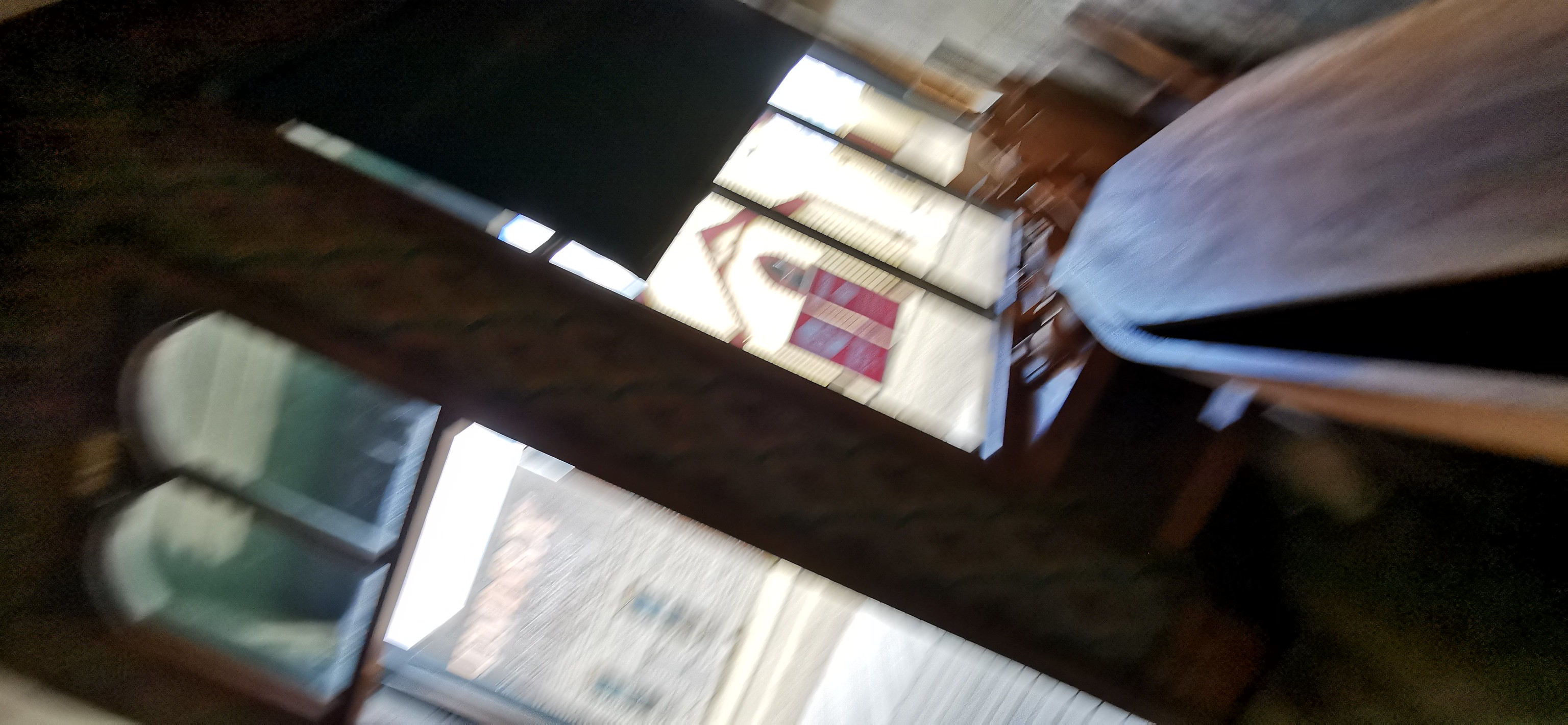The photograph is a blurred, tilted shot of the interior of a room, likely a small shop or store, looking outwards. The bottom of the image shows an open doorway with a long pane of glass. Above the door are two small, curved windows trimmed in dark brown wood, arranged in an M shape. Adjacent to these, on the left side of the image, are additional diagonal windows. The walls around the windows display a mix of green, white, and brown designs.

The room appears brightly lit, with a brown table in front of the center windows. To the right side of the image, there is an indistinct piece of furniture or wood against the wall, perhaps a dark wooden ledge. Outside the open door, there's a view of a small town area featuring a white building with red accents and another brick building with windows. The exterior also shows a beige structure with a visible roof and some kind of red sign. The image captures the feel of a quaint storefront, though the clarity is compromised by the blurriness and the angled shot.